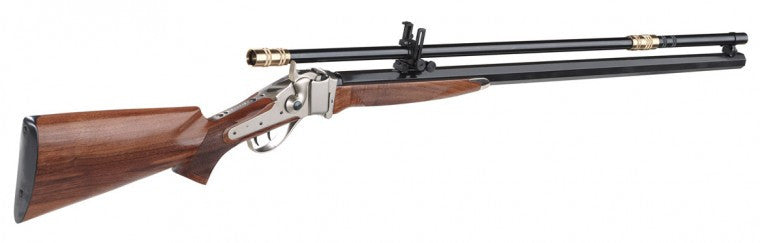The image features an older type rifle set against a completely white background, emphasizing the firearm itself. The rifle, facing towards the right with the right side visible, showcases a sleek design consisting of various materials and colors. The butt and handle of the rifle are crafted from a dark, shiny brown wood, leading up seamlessly to the metal components. The trigger and lever area is made from silver metal, highlighting intricate silver markings. The barrel, which is long and black, extends forward, with a metal rod on top—possibly a scope—adorned with gold color pieces that appear adjustable. The overall composition reveals a rifle in shades of black, silver, and brown, with additional detailing on the silver sections and the presumed scope, suggesting functionality and craftsmanship.